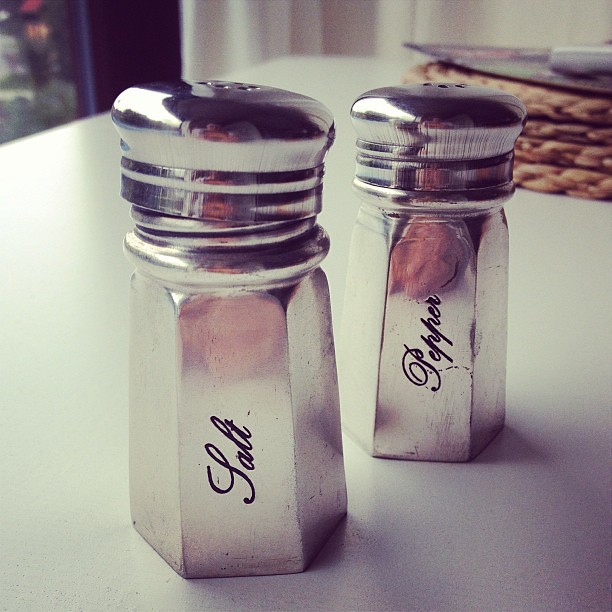This is a close-up color photograph showcasing a matching set of silver salt and pepper shakers with polished, reflective stainless steel surfaces. The salt shaker is positioned towards the front of the image, while the pepper shaker is slightly further back. Both shakers feature script lettering: "salt" written vertically on the salt shaker and "pepper" similarly inscribed on the pepper shaker. The salt shaker's chrome-colored screw cap is slightly ajar, whereas the pepper shaker's lid is securely fastened. The shakers are placed on a white table that has some visible scratches. In the upper right-hand corner of the background, a stack of round woven rattan or natural fiber placemats is visible, with an indistinct object on top. The reflective surfaces of the shakers hint at a vague reflection, adding depth to the image.